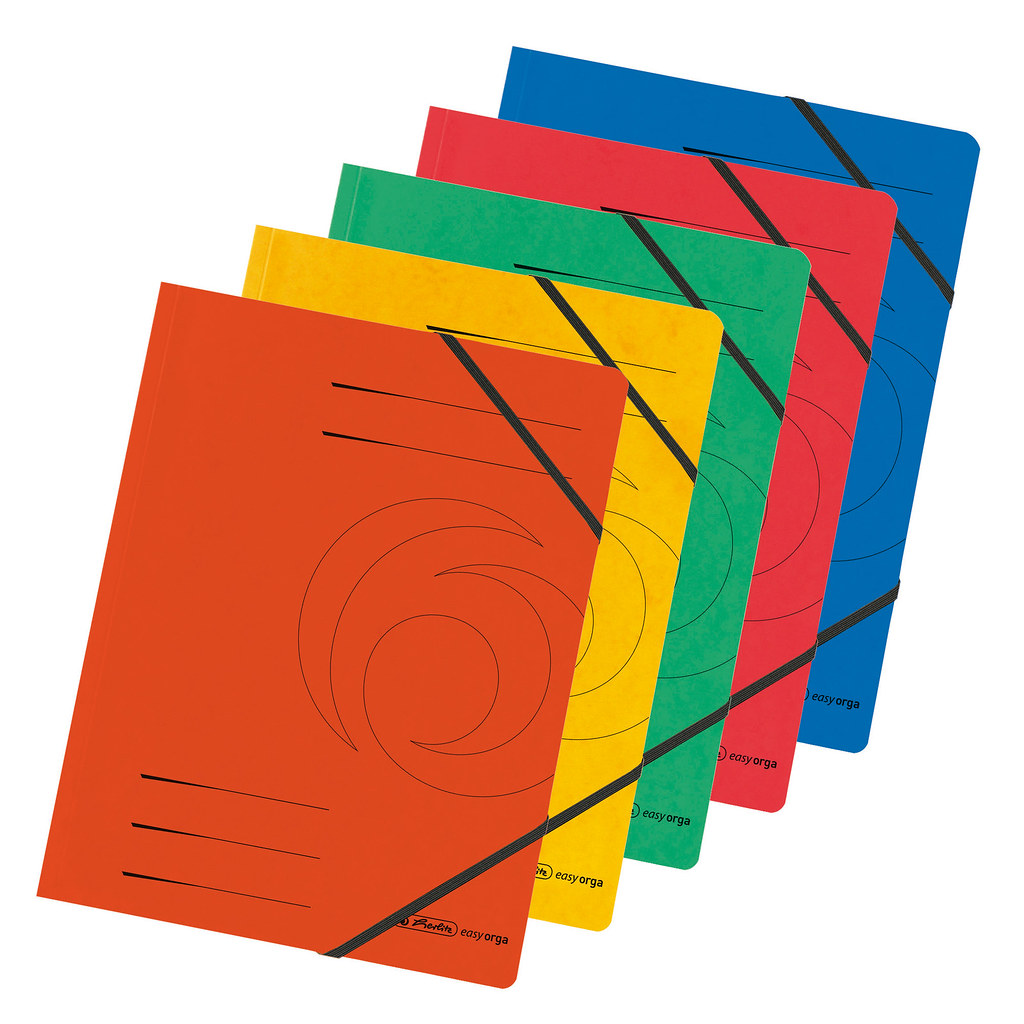This colored product image features a neatly stacked, diagonal arrangement of five rectangular sketch pads or notebooks. Each pad displays a unique color: orange at the front, followed by yellow, green, red, and blue. The notebooks overlay each other, creating a staggered effect that reveals a portion of each cover. Each cover is adorned with four or five horizontal lines and a crescent moon in the center, all outlined in pencil. The lower right corner of each pad features cursive lowercase text, spelling out "easy o-r-g-a." Additionally, black rubber straps stretch diagonally across the corners, contributing to a continuous black line effect along the bottom edges. The upper left and right corners of each notebook also have black diagonal stripes. The yellow notebook seems to have a textured appearance, with a variety of yellow hues interspersed across its surface. Binding along the side of each pad suggests their function as notebooks, reinforced by their design elements that could be used for labeling and organization.